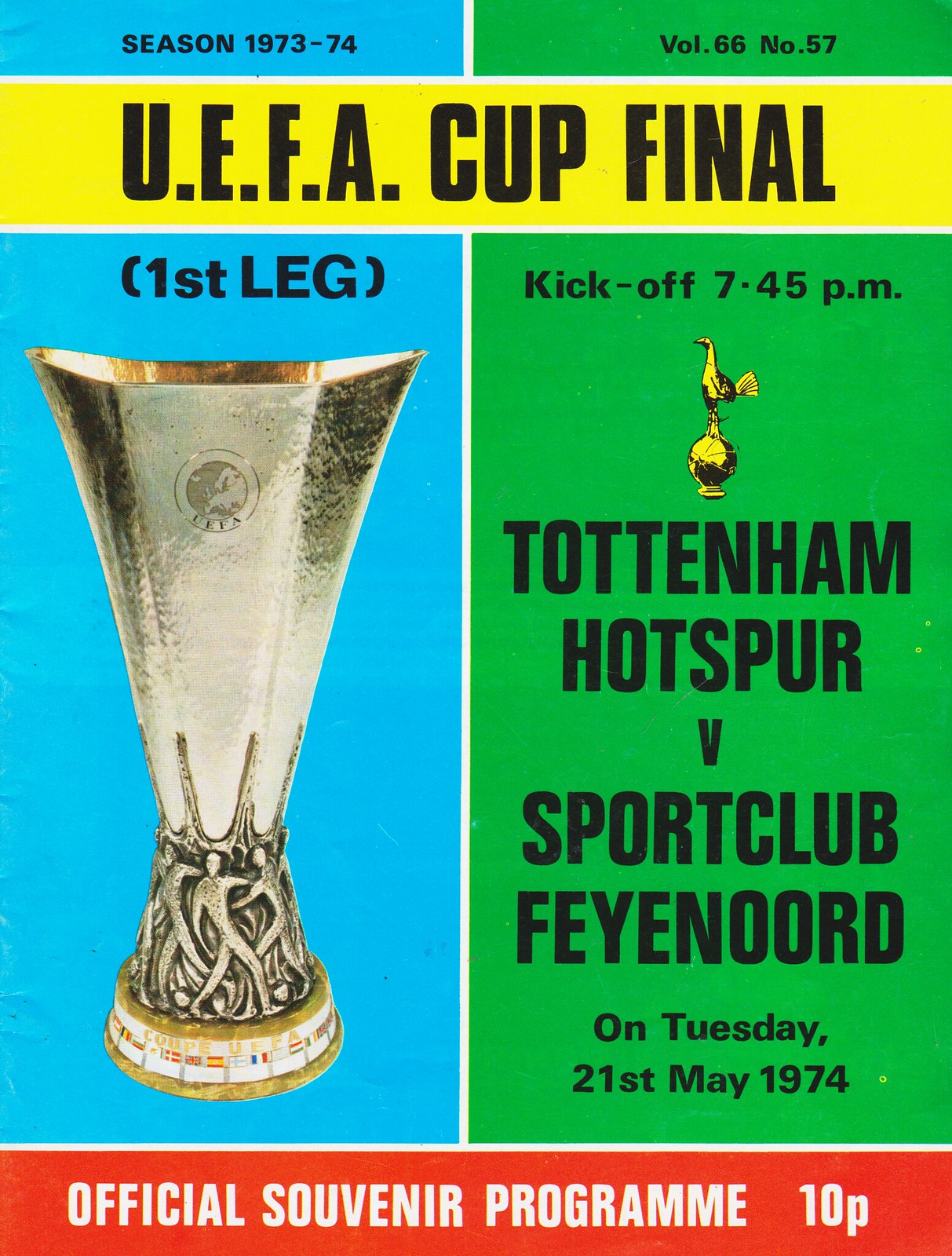This is the cover of an official souvenir program from the UEFA Cup Final held on Tuesday, May 21, 1974. The poster is divided into two parts: the left section is predominantly blue, and the right section is green. At the very top, a yellow banner spans both sections, indicating "UEFA Cup Final." In the upper left corner of the blue section, it says "Season 1973-74, Volume 66, Number 57" and below that, in brackets, it reads "First Leg." The blue section also features a large gold trophy that is octagon-shaped and vase-like, adorned at its base with various European country flags and figures of players holding it up. In the green section to the right, detailed information about the match is provided: "Tottenham Hotspur vs. Sports Club Feyenoord," with the kickoff time listed as "7:45 p.m." Additionally, at the bottom of the green section, the match date "Tuesday, 21st May 1974" is specified. A red banner at the bottom of the poster indicates the price, "Official Souvenir Program, 10 pence (10p)." The cover colors mainly consist of blue and green with accents in yellow and red, giving it a distinct and vibrant look despite its worn and tattered appearance.